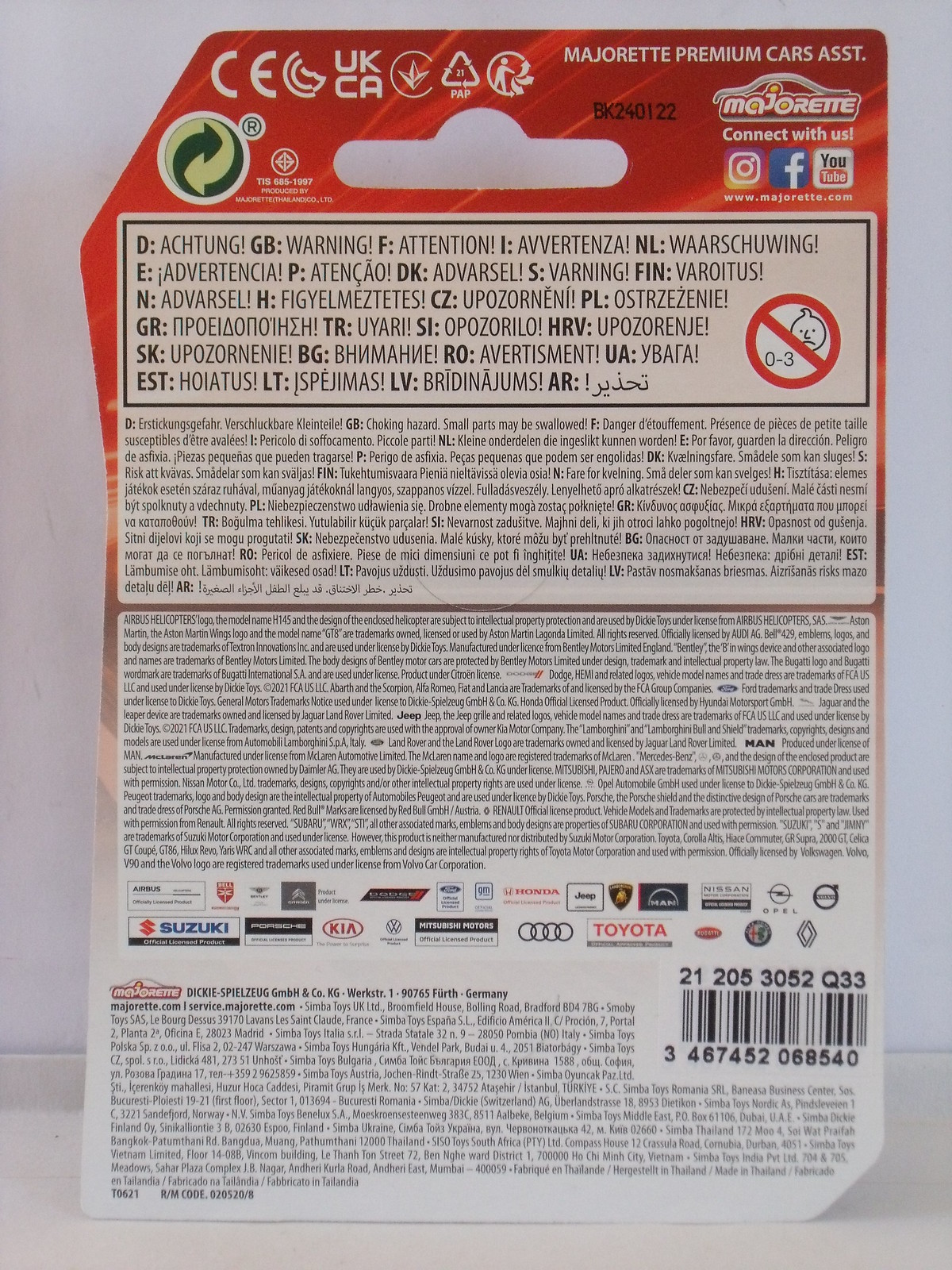This image depicts the backside of a toy car package. The package features a hang tab at the top for display on a store rack. Prominently displayed at the top center are the words "Majorette Premium Cars." Just below this title, there are icons linking to the brand's Instagram, Facebook, and YouTube pages. On the upper left corner, a small green recycling symbol can be seen. 

Numerous warning labels are scattered across the back, advising that the product is not suitable for children aged 0 to 3 years. These warnings are printed in multiple languages, with the text becoming increasingly smaller and harder to read, particularly for older individuals. 

Towards the bottom of the package, there are logos for several car brands including Suzuki, Toyota, and Kia. The bottom right corner features the package’s barcode. Overall, while it is evident that this is the back of a toy car package, the precise contents of the package are not clearly indicated.